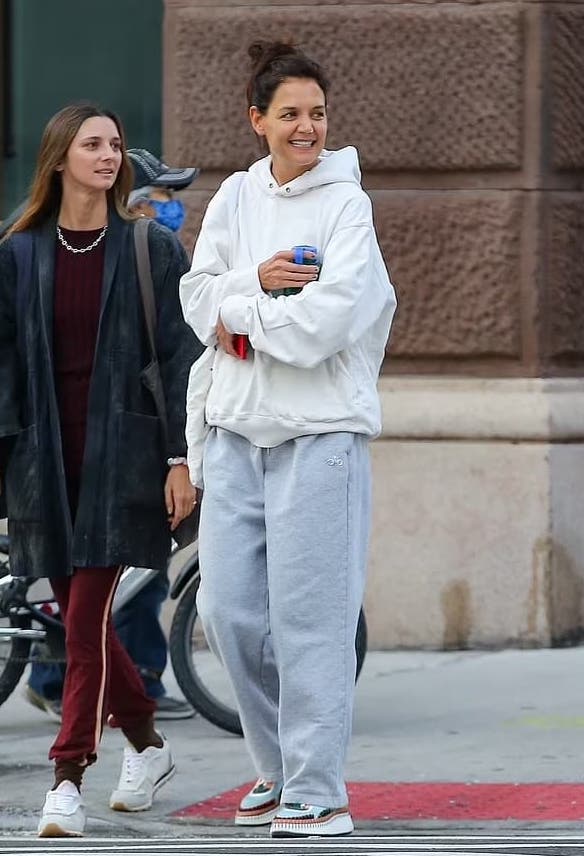This photograph, seemingly taken by paparazzi during daytime, features Katie Holmes prominently in the center, recognizable by her iconic look and style. Katie, the former wife of Tom Cruise, is casually dressed in a white long-sleeve hoodie, gray sweatpants, and stylish sneakers. Her dark hair is pulled back into a neat bun. She holds a phone in a red case in her left hand and a drink or bottled water in her right hand, although her crossed arms obscure both items from clear view. Standing to her right is another woman, who sports long brown hair cascading freely, with a youthful, slim appearance. She wears white sneakers, maroon jogger pants, a coordinating maroon top, and a black, thigh-length coat, accessorized with a silver necklace and bracelet. Both women appear to be white and are standing on a city sidewalk, gazing into the distance. The background reveals a slightly blurred building with a distinctive green-white lower section and a chocolate brown upper section featuring large brick patterns. An old cyclist, masked and capped, is faintly visible between the buildings and a green-colored structure, contributing to the urban atmosphere.